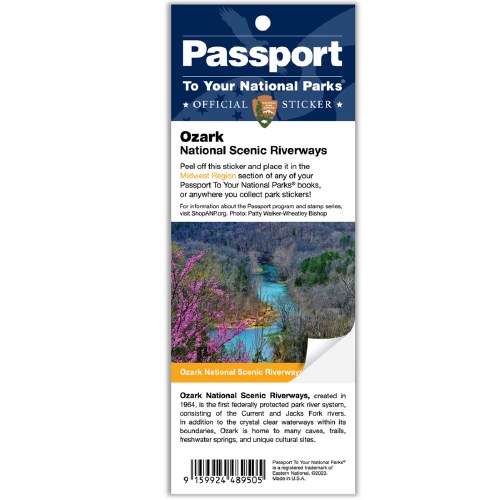The image is a rectangular official sticker for a national park, specifically designed for collectors of national park memorabilia. At the top of the sticker, against a blue background, the text "Passport To Your National Parks" is prominently displayed in white. Just below, "Official Sticker" is written, with the crest for Ozark National Scenic Riverways situated between the words. Above "Passport," there is a distinctive white circle.

Further down, the text "Ozark National Scenic Riverways" appears, instructing users to peel off the sticker and place it in the Midwest region section of their "Passport to Your National Parks" book or wherever they collect park stickers. This instructional text is set against a clean white background.

The lower portion of the sticker features a photograph of the Ozark National Scenic Riverways, characterized by a picturesque river flanked by lush, green, and some purple-hued trees. Notably, the bottom right corner of the photograph gives the impression of peeling off, adding a dynamic element to the design.

At the very bottom, additional text provides historical context about the Ozark National Scenic Riverways, noting its establishment in 1964 as the first federally protected park river system. Adjacent to this information is a barcode accompanied by fine print. The entire rectangular image has a subtle shadow, giving it a slight lift from the background.